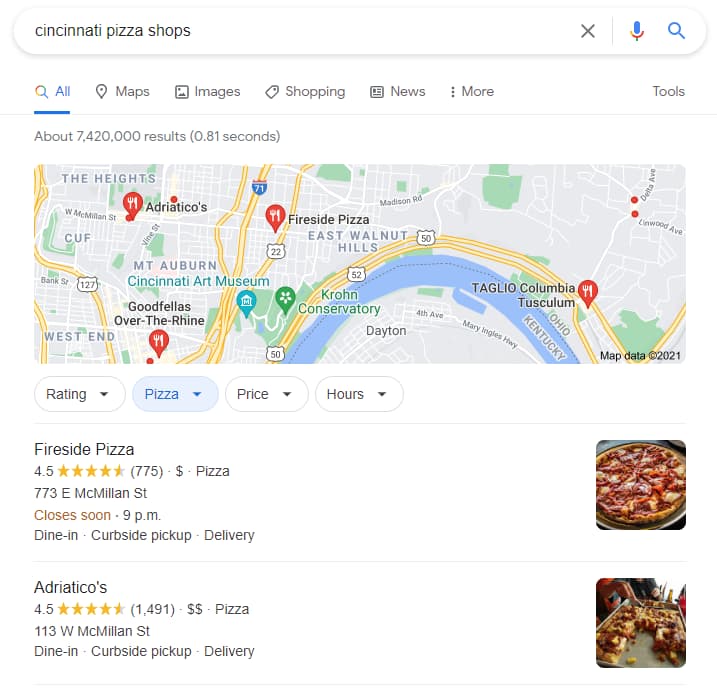A Google search for "Cincinnati Pizza Shops" displays at the top of the screen, showing 7,420,000 results in 0.31 seconds. The search options include categories like All, Maps, Images, Shopping, News, More, and Tools. Below it, a map of Cincinnati highlights four different locations marked by red location pins. The surrounding areas mentioned on the map are The Heights, West End, Mount Auburn, East Walnut Hills, Cincinnati Art Museum, and Krone Conservatory. 

Beneath the map, the first listed result is "Fireside Pizza," rated 4.5 stars with 775 reviews. It is categorized under Pizza with a single dollar sign ($) and is located at 773 East McMillan Street. The restaurant is noted for offering Dine-In, Curbside Pickup, and Delivery services, and it closes soon at 9 p.m.

The next result is "Adriatico's," also rated 4.5 stars but with 1,491 reviews. This pizza place falls under the $$ category and is situated at 113 West McMillan Street.